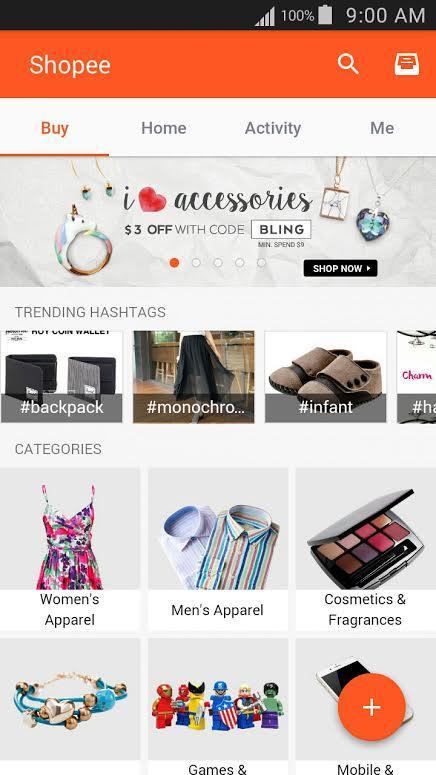This screenshot is from a mobile phone displaying the Shopee app interface. The screen has a thin black header indicating a full battery at 100% and displaying the time as 9:00 AM. Below this, an orange header bar prominently features the Shopee logo on the left and a search icon along with an unspecified square icon on the right. 

The interface is divided into four main tabs: 'Buy,' 'Home,' 'Activity,' and 'Me,' with the 'Buy' tab highlighted in orange, denoted by an orange line underneath it. 

At the top part of the 'Buy' section, there's an advertisement for iHeart accessories, showcasing images of jewelry with buttons labeled "Bling" and "Shop Now." Below this ad, a section titled "Trending Hashtags" appears, though the last hashtag is partially cut off. The visible hashtags include #backpack, #monochrome, and #infant, each accompanied by corresponding photos.

Further down, the 'Categories' section is displayed with six square items set against a very light gray background, featuring images and labels. The categories listed are:
- Women's Apparel
- Men's Apparel
- Cosmetics and Fragrances
- Jewelry (unnamed)
- Games
- Mobile Accessories (partially named)

Notably, the sixth square depicts a mobile phone, partially overlaid with an orange circle containing a white plus sign.